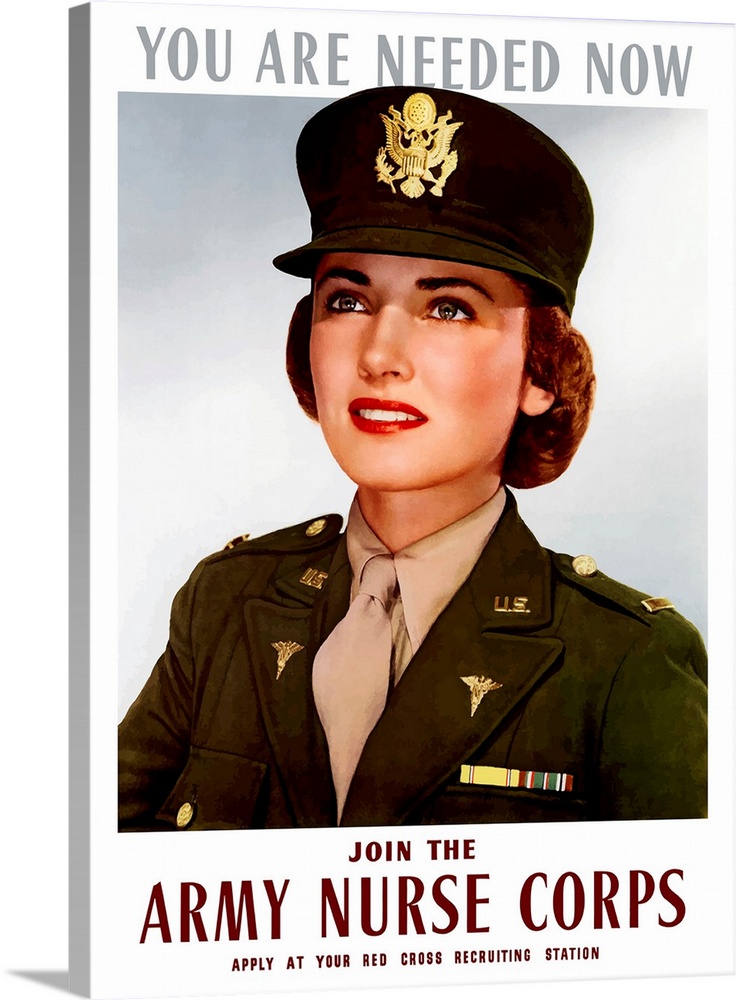This World War II era poster features a striking image of a woman proudly wearing an Army Nurse Corps dress uniform. The poster has a white background with a large, colorful photograph of the woman at its center. She has dark brown hair neatly collected at the nape of her neck, and she wears an olive green cap adorned with a gold eagle emblem in the front. Her makeup is striking with bright red lipstick, and her blue eyes stand out against her pristine white teeth. The woman is dressed in an olive green jacket over a beige shirt and tie, and on each lapel of the jacket, she sports a gold brooch. 

Above her head, the poster reads "You are needed now" in gray letters, while beneath her picture, in brown letters, it says, “Join the Army Nurse Corps. Apply at your Red Cross recruiting station.” This vintage advertisement vividly illustrates the essential and honorable role women played during World War II, drawing attention both for its historical importance and its call to action.